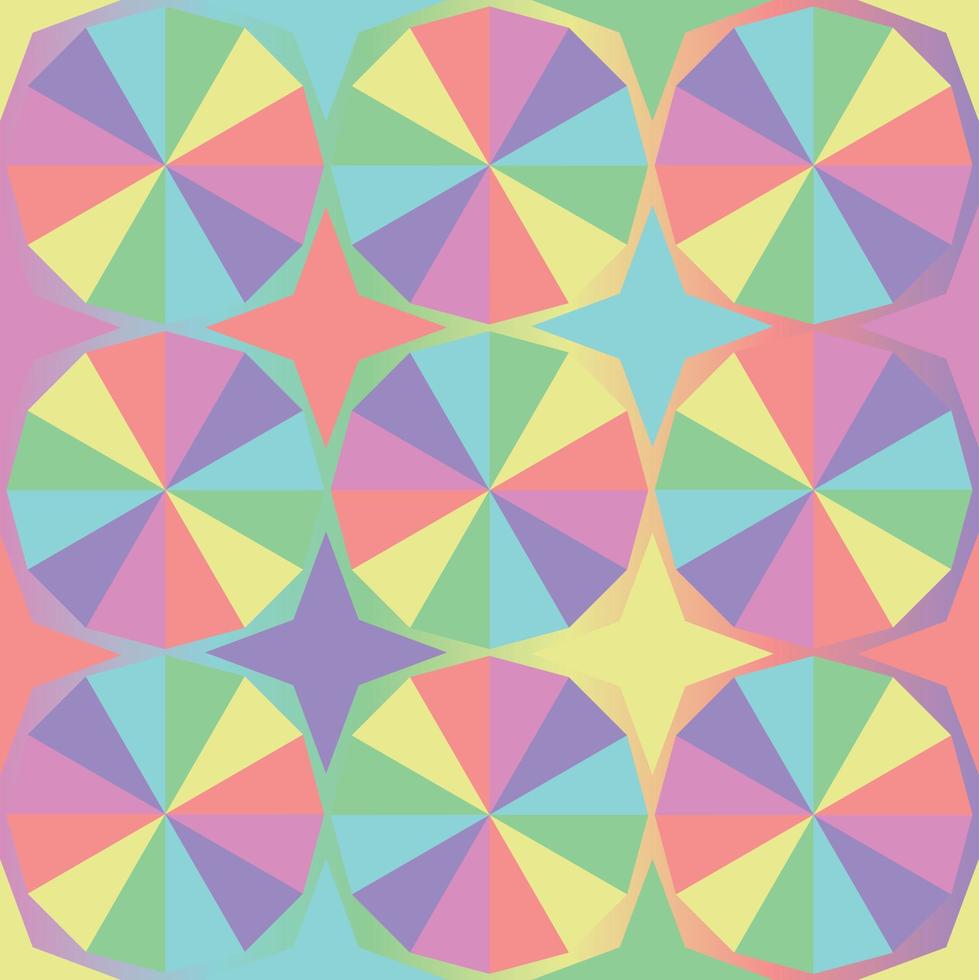This image appears to be a vivid and colorful illustration, potentially created with watercolor or graphic design elements. It features nine circular shapes arranged in a 3x3 grid, each resembling a top-down view of umbrellas. These circles are intricately divided into wedge-like slices, reminiscent of pizza slices, and each slice is painted a different color, forming a spectrum that includes red, yellow, green, blue, violet, purple, orange, pink, and aqua hues. Connecting these circles are star-like elements filling the gaps between them; of these, four prominent stars are central and distinct in color—red, blue, yellow, and purple. The entire composition is awash with vibrant yet soft shades indicative of watercolor, creating a harmonious blend of colors that spread across the background and the shapes themselves, suggesting a whimsical, finished feel suitable for a magazine cover or an artistic coloring book page.